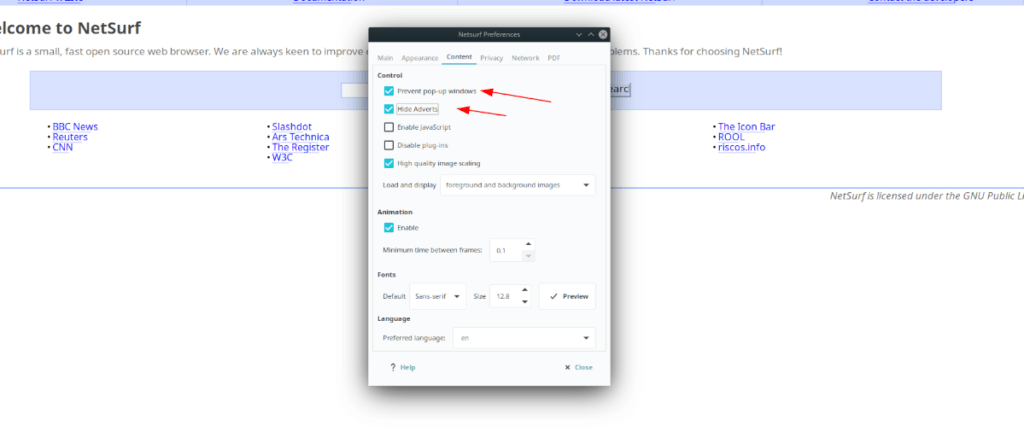The image is a left-to-right horizontal screenshot, likely from a computer or smartphone. The background is predominantly white, akin to a default screen. At the top of the screen, a long, purple line stretches horizontally, featuring alternating sections of darker and lighter purple hues. In the upper left-hand corner just below this line, bold black text reads, "Welcome to NetSurf," although the "W" and "E" in "Welcome" are cut off.

Below, there is a sentence that is partially obscured by a prominent rectangular pop-up box in the center of the screen. Despite the obstruction, we can observe a long purple rectangular box with some text within it on the background. Below this, there are several clickable links in blue, displayed in bullet points: BBC News, Reuters, CNN, Stash.ArtsTechnica, The Register, W3C, the icon bar, rule, and riscos.info.

The central focus of the image is the pop-up box labeled "NetSurf Preferences" at the top in a black bar. Within this box, a set of clickable icons is displayed: Main, Appearance, and Content (which is bolded and underlined), Privacy, Network, and PDF. Below these icons, there are several control options with selected checkboxes: "Prevent pop-up windows" and "Hide adverts," each accompanied by red arrows. The checkboxes for "Enable JavaScript" and "Disable plugins" are not selected. Additional settings for "Animation," "Fonts," and "Language" are also available for customization.